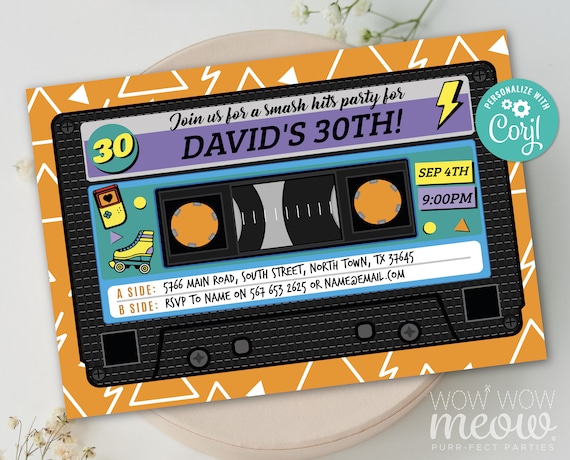Displayed on a white table or counter, this vibrant birthday invitation lies atop a couple of white plates surrounded by dried baby breath flowers. The invitation, themed around a nostalgic VHS tape, has an orange background adorned with white triangles and lightning bolts. The center of the card mimics a vintage cassette tape, featuring a black tape design. Prominently, a green circle with the number 30 in yellow is displayed on top, surrounded by a purple and dark purple border. The card enthusiastically invites you to "Join us for a smash hits birthday for David's 30th," highlighted by a striking yellow lightning bolt. The bottom section of the card is blue, showcasing a roller skate and a Gameboy graphic. Key details include the date "September 4th" in yellow and black, with the time "9 p.m." in purple and black. A white strip at the bottom reads "Side A: 5766 Main Road, South Street, North Town, Texas 376545" and provides RSVP details, including a phone number, "561-653-2625," and an email address. Additionally, there's a blue circle in the top corner and a label at the bottom right stating "Personalized with Coral," finished off with the quirky tagline "Wow Wow Meow Perfect Parties." This invitation blends a playful retro aesthetic with detailed event information, making it a unique keepsake.